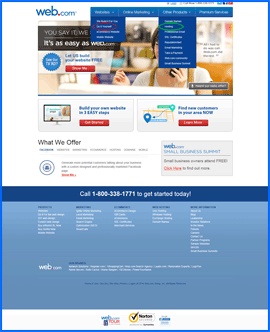A small screenshot of a website named "web.com" is displayed. The website's title is prominently positioned at the top left corner. To the right of the title, a series of drop-down menus are aligned horizontally, all set against a navy blue background. The backdrop of the site features a stock image of a woman holding up a phone, adding a personal touch to the interface. Scattered around the image are various descriptive texts and several small red buttons, likely for navigation or calls to action. The web design appears clean and functional, with a focus on clarity and ease of use.